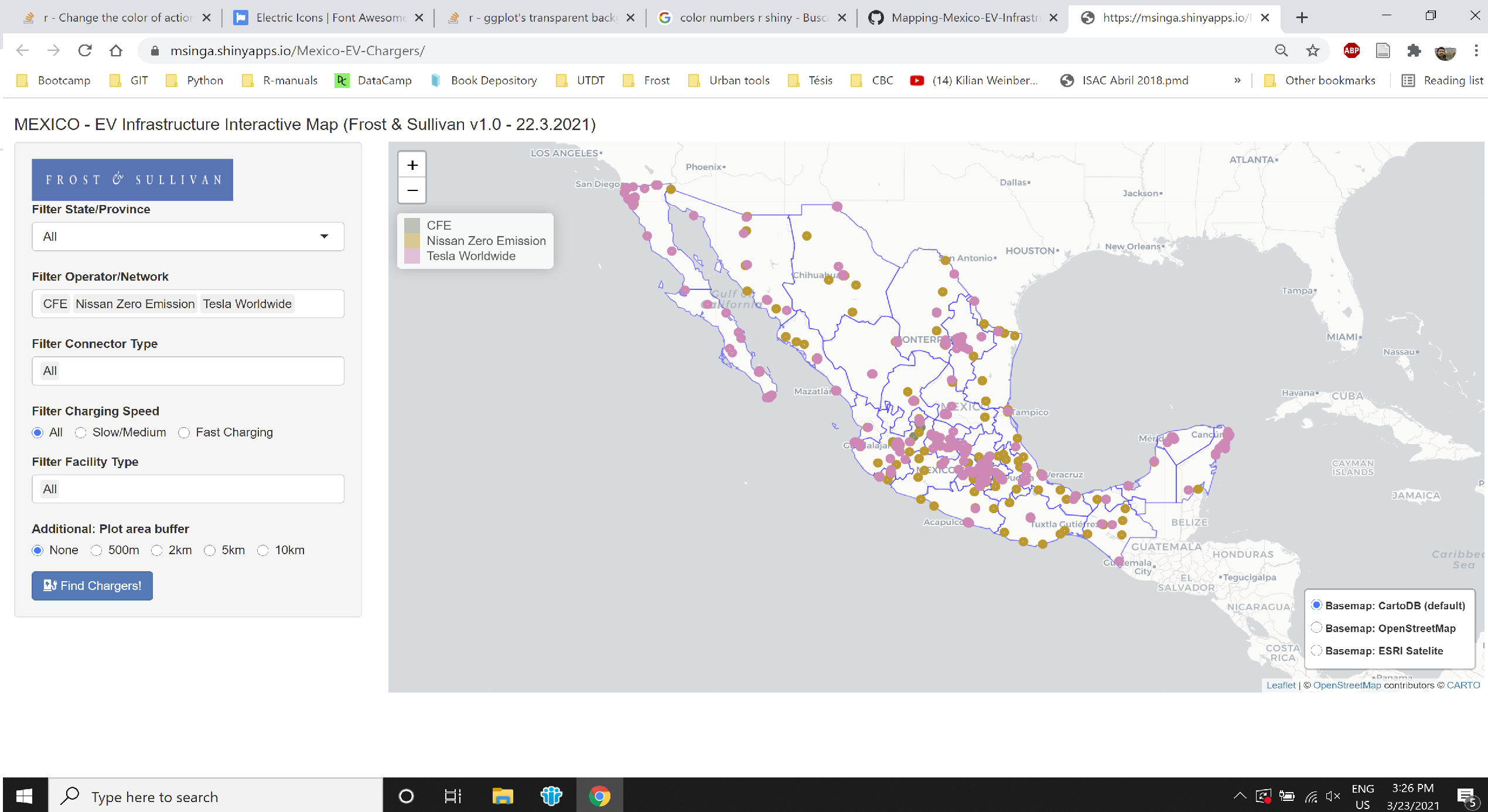This detailed screenshot captures a desktop web browser interface, providing a clear view of the user's browsing environment. At the top, a light gray background accommodates six browser tabs. The first five tabs, which are not selected, each feature an icon on the left, followed by a title in medium gray text, and a vertical light gray line separating each tab. Their titles, partially cut off, read as follows:

1. "change the color of Aksha"
2. "electric icons, font awesome"
3. "ggplots transparent back"
4. "color numbers are shiny, R-BUSC"
5. "mapping Mexico EV infrastructure"

The sixth tab, which is selected and marked by a more white background, displays the beginning of a URL: "https://msinga.shinyapps.io/".

Directly below the tabs, the browser's URL bar with a light gray background and rounded ends is shown. A medium gray lock icon appears on the left, with the text "msinga.shinyapps.io/Mexico-EV-chargers/" to the right of it.

The content below that consists of a white header featuring various icons and their corresponding titles, mainly depicted as manila folder icons paired with text. The titles from left to right include:

- Bootcamp
- GIT (all caps)
- Python
- R-manuals
- Datacamp
- Bookdepository
- Utdt
- Frost
- Urbantools
- Tesis (with an accent on the 'e')
- Cbc
- Killianweinberg...
- Isacabriel2018.pmd
- Other bookmarks
- Reading list

Beneath this header is a detailed map of Mexico, marked with numerous pink dots and interspersed with squiggly blue lines that delineate the different states.